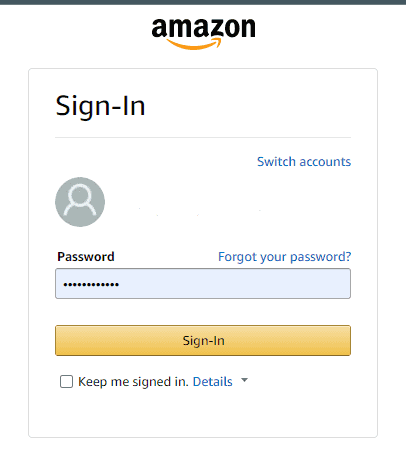The image showcases the Amazon sign-in page. 

At the very top, there is a thin black line. Centered below, the iconic Amazon logo features the word "Amazon" with its distinctive orange smile. The entire background of the interface is gray.

Beneath the logo, there is a prominent rectangular sign-in form bordered by a thin gray line, taller than it is wide. The bold black text "Sign-In" is the largest font on the page and is located at the top of the form. 

A thin gray line separates this from the elements below. On the right, in blue text, is the "Switch accounts" option, and on the left is a circular icon with a generic avatar.

Further down, the word "Password" appears in black, with the "Forgot your password" link in blue on the right. Below this, a password input field shows obscured data (dots) within a blue and gray-bordered box.

Following the input field, the yellow sign-in button takes up the same width, featuring the text "Sign-In" in black. 

Beneath the button, there is a checkbox labeled "Keep me signed in," with the "Details" link in blue and a drop-down arrow. The checkbox is not selected, and the background here remains white.

The color palette of the entire page includes shades of black, white, yellow, various blues (both dark and light), orange, and gray.